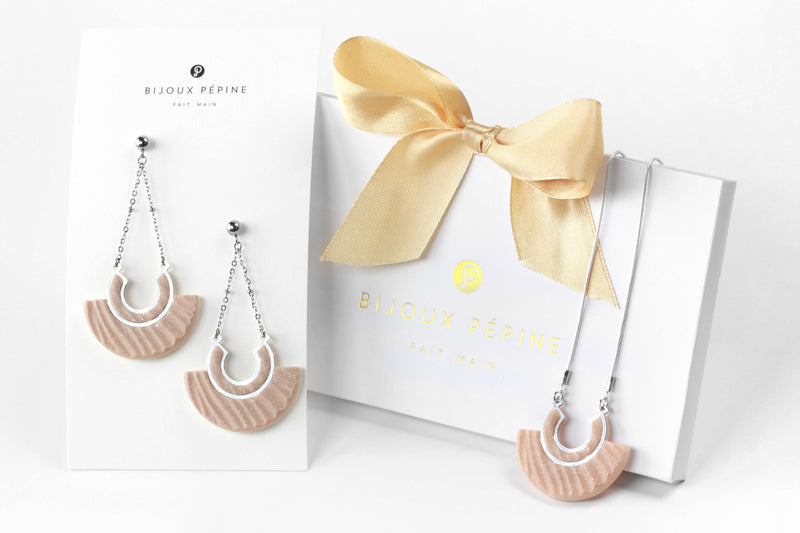The image showcases an elegant jewelry set by Bijou Pepin, prominently displayed on an off-white background. The left side features a rectangular white card with two long, dangling earrings. These earrings consist of silver chains descending into a fan-shaped pendant with a pale peach color and a white border. On the right side, a matching necklace drapes elegantly over a white jewelry box adorned with a pale yellow bow. The box, featuring the text "Bijou Pepin" in shiny gold that is slightly difficult to read, also carries the brand's logo— a yellow circle with a white, ornate "P" in its center. The sophisticated design and consistent color scheme of peach and white, paired with silver accents, make this jewelry set the focal point against the minimalist background, suggesting a studio setting intended for advertising.